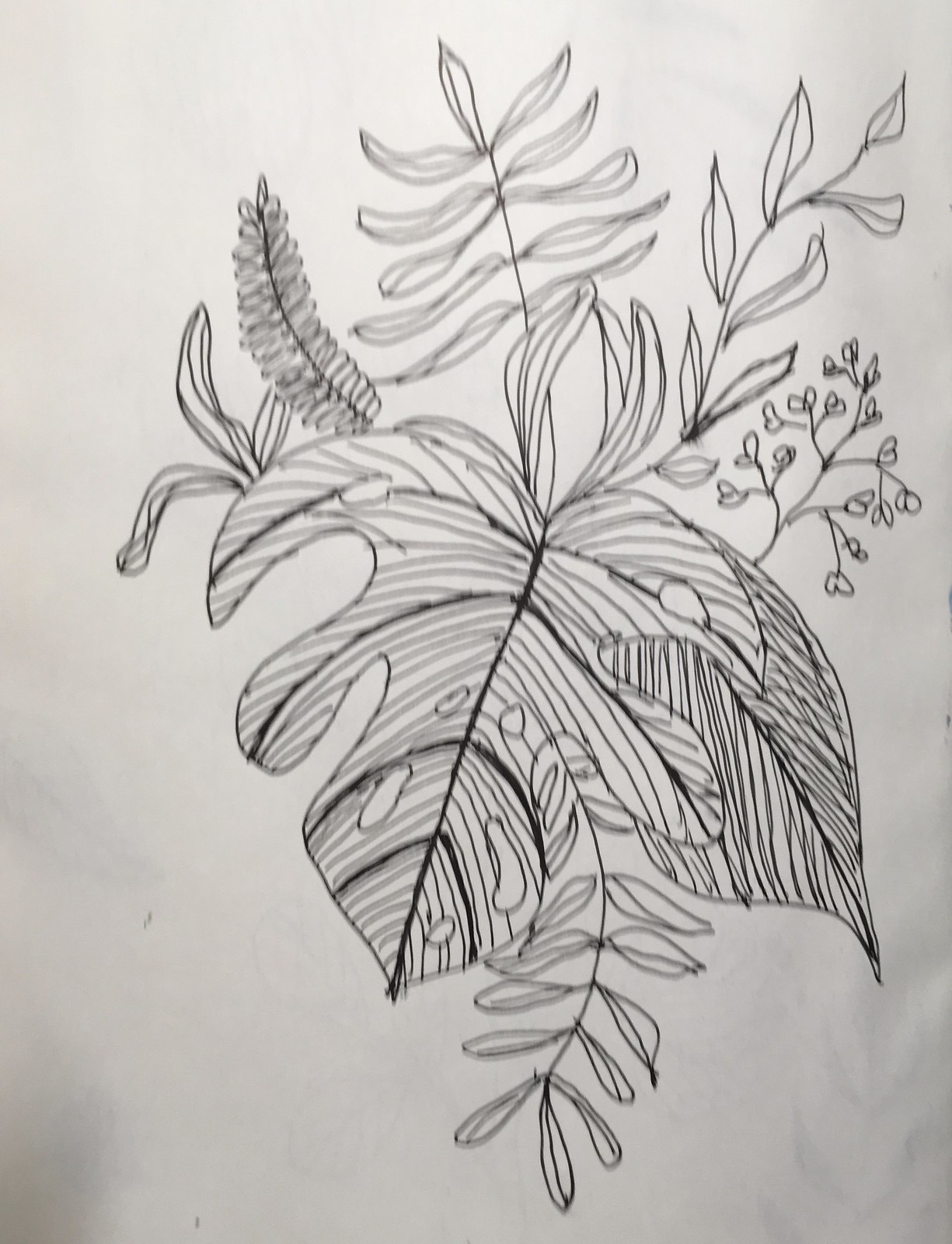This detailed pencil and black colored pencil drawing, set against a whitish-gray, thin sketch pad paper, showcases an intricate arrangement of leaves and twigs. The centerpiece is a large, oak-like leaf with a pointed base and four rounded sections on top, darkened lines accentuating its veins and stem. Attached to a thin twig, this primary leaf is accompanied by smaller, round leaves along the twig's length, and identical pairs of leaves at the top. Additionally, two other types of twigs feature small, heart-shaped leaves. The background reveals subtle shadows and faint hints of another illustration, adding depth to this meticulously crafted artwork.